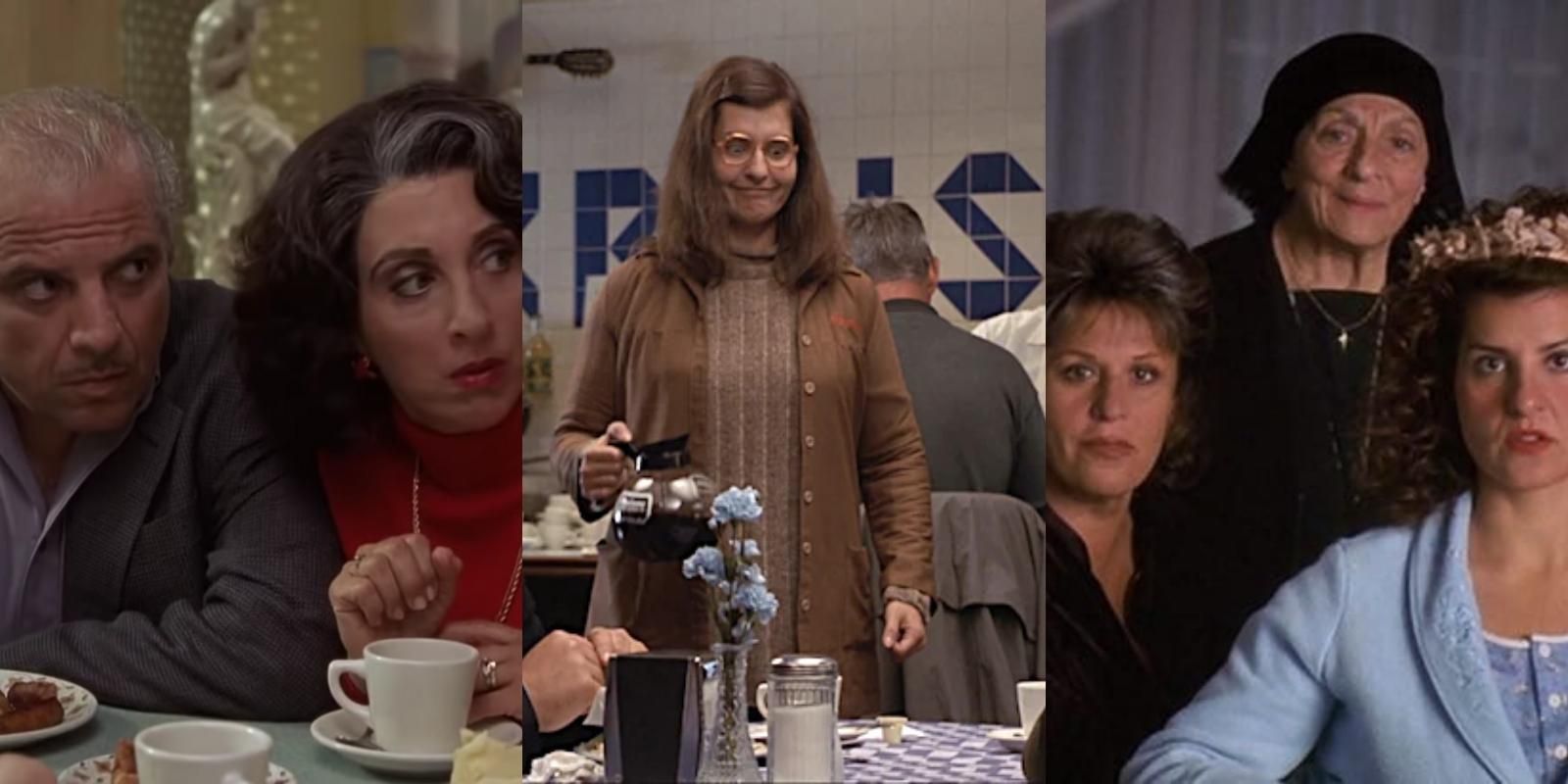The image is a vertically divided triptych, each section depicting scenes reminiscent of "My Big Fat Greek Wedding." On the left, an older couple, possibly in their 50s or 60s, are seated at a diner table, both gazing intently to the right. The man has gray hair while the woman sports bushy brown hair with a gray streak. The middle section features a middle-aged woman with glasses and brown attire, holding a coffee pot, standing next to a diner table adorned with flowers, a napkin holder, and a sugar jar. The right section presents three women arranged in a triangular formation; an elderly woman in a black head covering and dress stands at the back, while in front, a slightly younger woman, around 50 years old, sits to the left, and a younger woman, approximately 35-40 years old, dressed in blue with a golden wreath on her head, sits to the right. The scene is set with muted tones of gray, blue, yellow, red, and brown, and features some indistinct text on the wall tiles in the background.